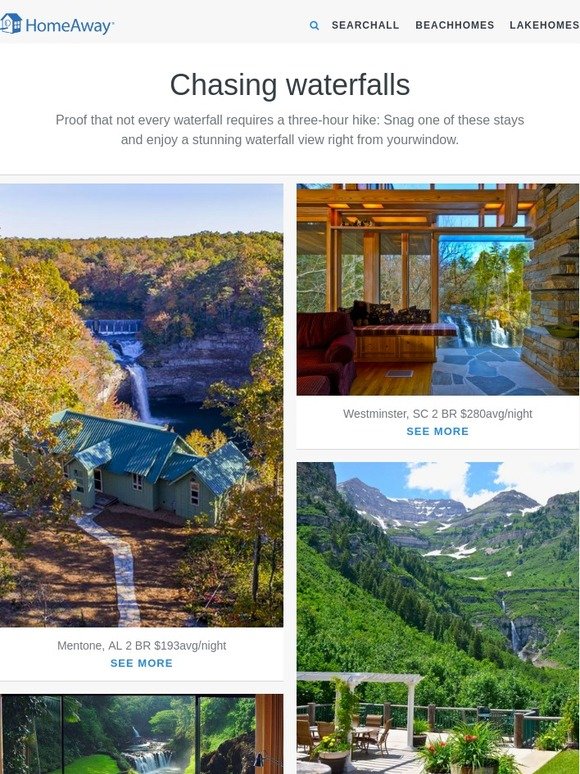The image depicts a webpage from "HomeAway" – a vacation rental platform. At the top left corner, the "HomeAway" logo, consisting of a blue house icon and the name "HomeAway" in blue text, is prominently displayed. On the top right corner, various categories are listed: "Search All," "Beach Homes," and "Lake Homes," with a blue magnifying glass icon to the left of "Search All."

Beneath the top navigation, in the central section, is a banner featuring the phrase, "Chasing Waterfalls." The subtitle reads, "Proof that not every waterfall requires a three-hour hike. Snag one of these stays and enjoy a stunning waterfall view right from your window."

Below this banner, several images showcase picturesque rental properties adjacent to waterfalls. On the middle left, an image presents a lush green and yellow treescape with a blue-colored house at its center, backed by a waterfall. The caption underneath reads, "Mentone, AL, 2BR, $193 average per night." To the right of this image is another showcasing a verdant area with a striking blue waterfall.

The overall aesthetic of the page is inviting and serene, promising potential renters beautiful views of natural waterfalls right from their accommodations.